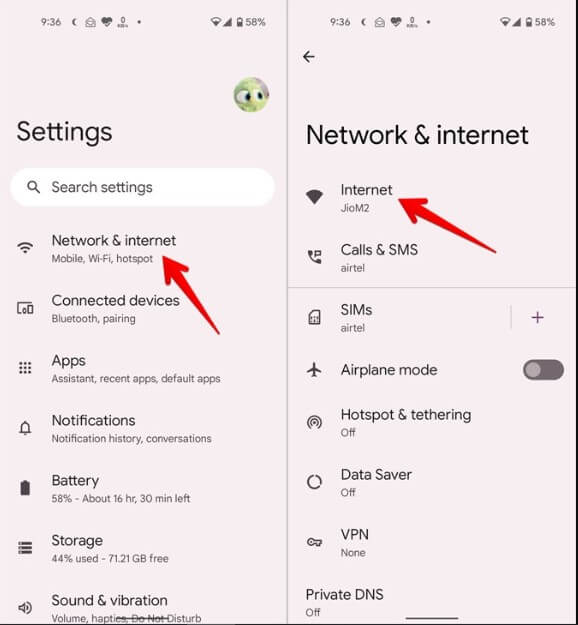**Smartphone Settings Navigation: Network and Internet**

In the first screenshot, taken from a smartphone, the time displayed at the top of the screen is 9:36, accompanied by various standard icons found within the settings menu. The primary section visible on the screen is the "Settings" page, prominently titled at the top. Directly below the title is a search bar for quickly locating specific settings.

Below the search bar, the main categories of the settings menu are listed sequentially as follows:
1. Network & Internet
2. Connected devices
3. Apps
4. Notifications
5. Battery
6. Storage
7. Sound & vibration

A red arrow explicitly points to the "Network & Internet" option, indicating it is the focal point of this step.

In the subsequent screenshot, the settings have been navigated to the "Network & Internet" section. Here, another red arrow directs attention to the "Internet" category at the top of the list, confirming an active internet connection with the icon marked in solid black. Beneath "Internet," the "Calls & SMS" section is visible, followed by "SIMs." The SIM card is identified as "Airtel," and alongside it, there is a toggle option indicated by a plus arrow icon, which can be switched on or off. The final visible setting in this screenshot is "Airplane mode."

Through these detailed steps, the screenshots illustrate the navigation process within the smartphone's settings to access network and internet-related options.